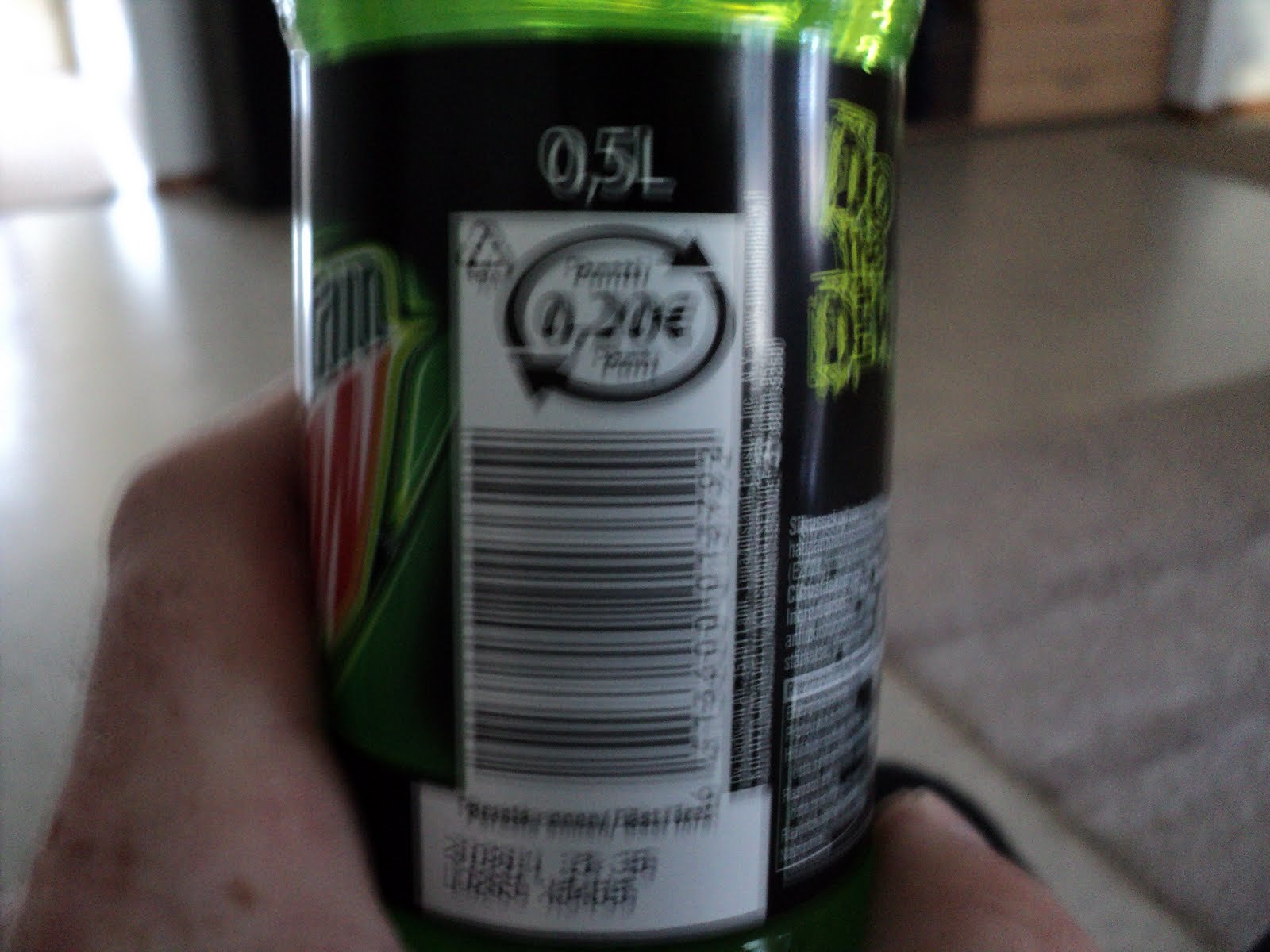A close-up photograph features a fair-skinned individual holding a green transparent plastic bottle of Mountain Dew soda. The person's hands, adorned with either liver spots or freckles, prominently display the bottle's barcode and product information. The label boasts a black background with white fields and the iconic Mountain Dew logo. The bottle contains 0.5 liters of the vibrant soda.

In the background, a variety of textures and details are visible: a beige rug on one side, a shiny floor surface, and a darker brown rug partially seen in the distance. A set of horizontal wooden dresser drawers adds to the domestic setting, against white walls with medium brown floor trim. Sunlight filters into the scene, suggesting the photo was taken during daytime, adding a warm, natural light to the image.